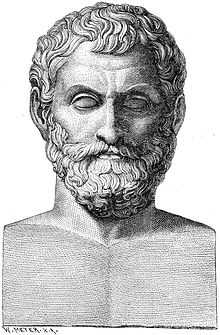This is a detailed black and white illustration, resembling a pen and ink drawing, of a classical bust depicting a Roman or Greek figure, possibly an emperor, philosopher, or poet. The bust, with its grayish or silverish tones, showcases the upper torso of the man, who appears to be bare-chested. His hair, which is curly and styled forward, complements a thick beard and mustache that frames his face closely. The subject's eyes are closed or without pupils, accentuating a thoughtful demeanor. A slight crease marks the forehead, hinting at contemplation or wisdom, characteristics often associated with iconic figures like Marcus Aurelius or Virgil. The signature of the artist is present in the lower left-hand corner, but it is too small to decipher. This intricate illustration captures the essence of a revered individual from the classical world, emphasizing both the intellectual and aesthetic attributes typical of such historical representations.